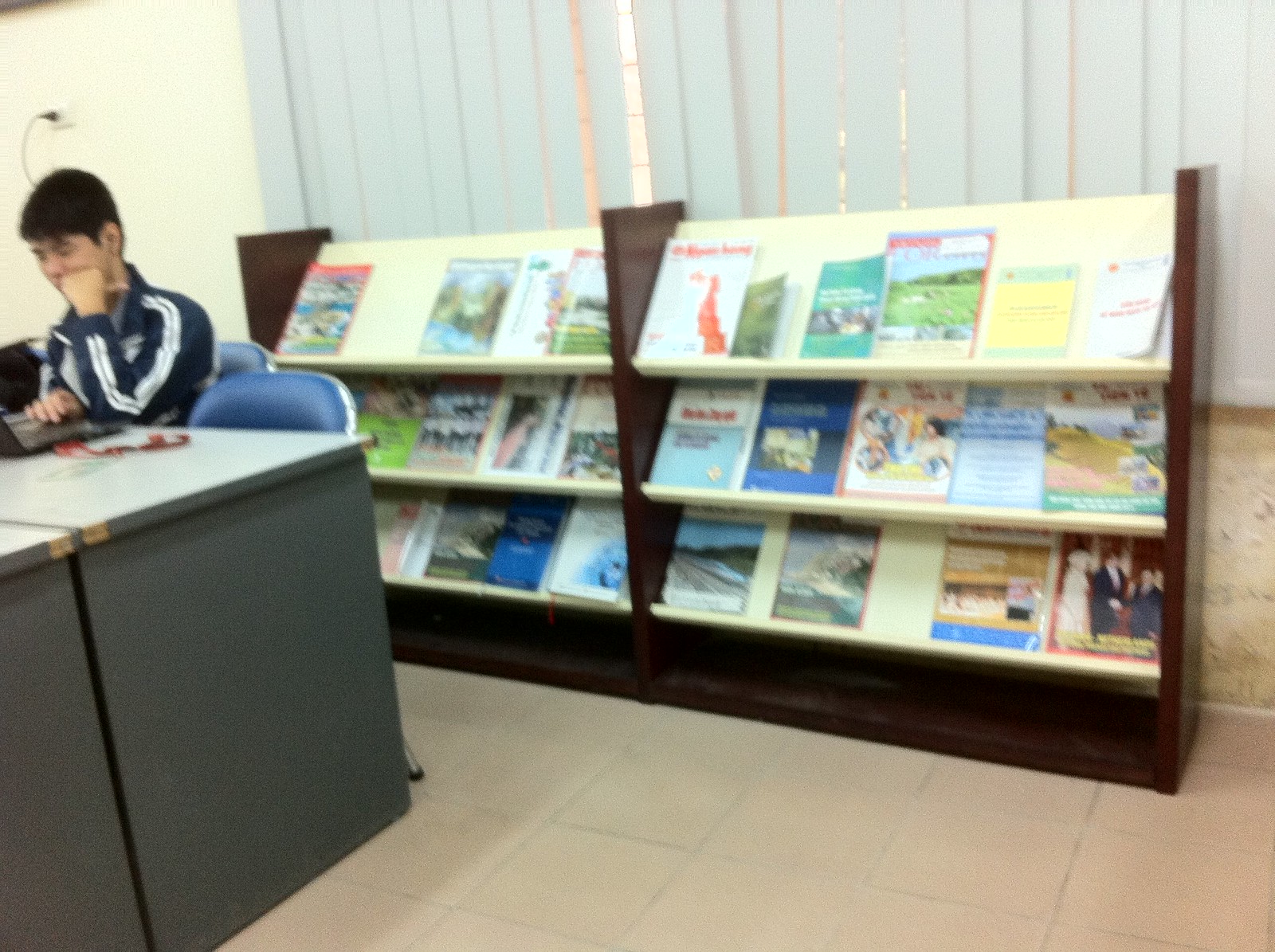In this image, a young man, possibly a high school student, sits at a gray table in a library. He is wearing a blue tracksuit with white stripes and has dark black hair. His hand rests on his cheek as he concentrates on a gray laptop in front of him. The chairs at the table have metal frames with blue backrests. To his left, there is an empty seat. Behind him, a wooden magazine rack with a yellow backing occupies the wall. The magazine rack is divided into two sections with a wooden center divider and three angled white shelves, which display a variety of multicolored magazines and booklets. Above the rack, there is a window with a blue slatted curtain. The library's floor is tiled in a tan color.